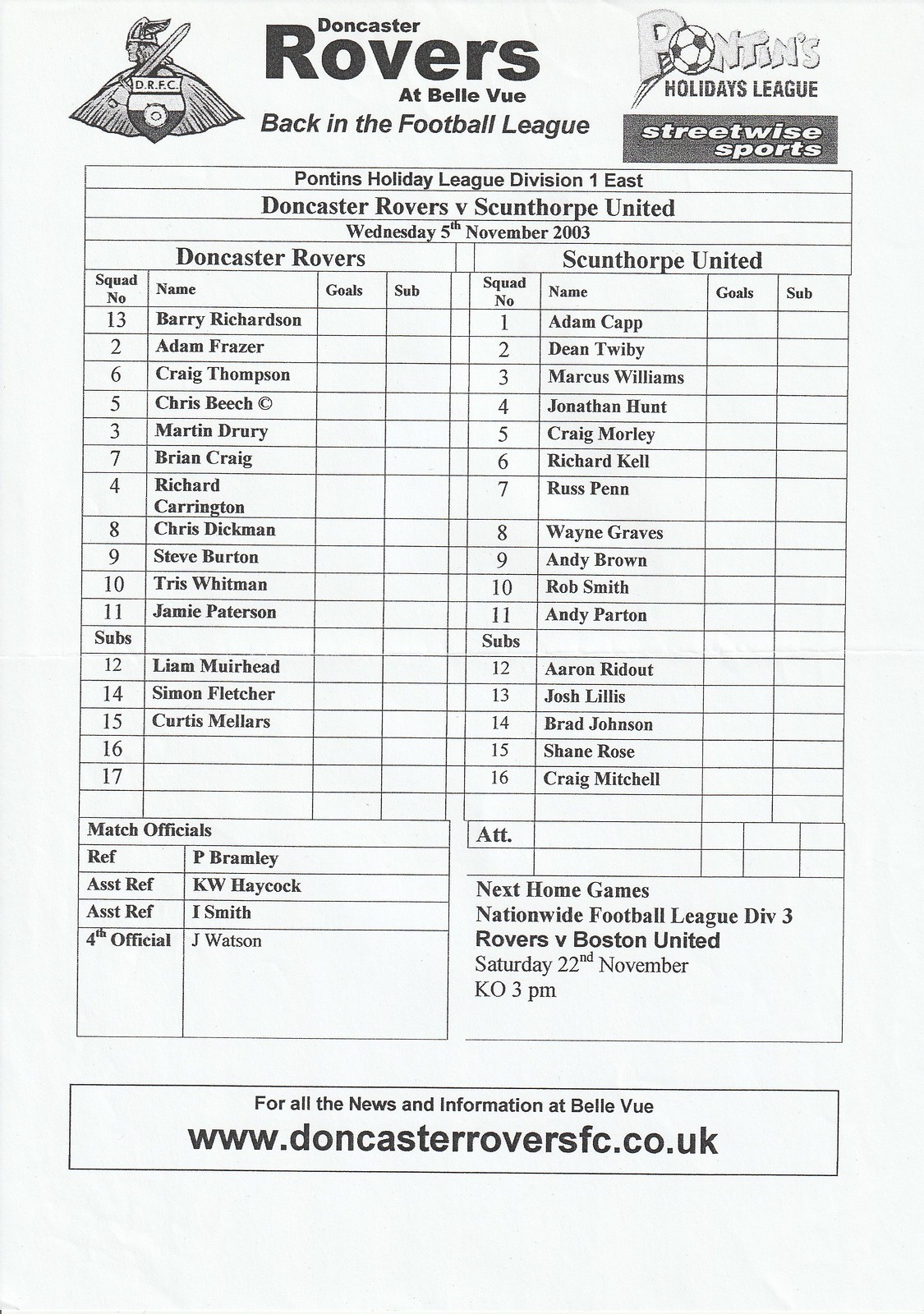This image features an official roster for a soccer game held at Bellevue, detailing a matchup between Doncaster Rovers and Scunthorpe United in the Pontins Holidays League Division 1 East. Dated Wednesday, November 5, 2003, it prominently displays a grid listing approximately 13 players for each team, with Doncaster Rovers on the left and Scunthorpe United on the right. The top of the document proudly announces "Doncaster Rovers at Bellevue, back in the football league." The Doncaster Rovers' emblem is positioned at the top left, while the logo for the Pontins Holidays League is at the top right alongside the "Streetwise Sports" insignia. Additional details at the bottom of the document direct readers to visit doncasterroversfc.co.uk for more news and information about Bellevue and the team.